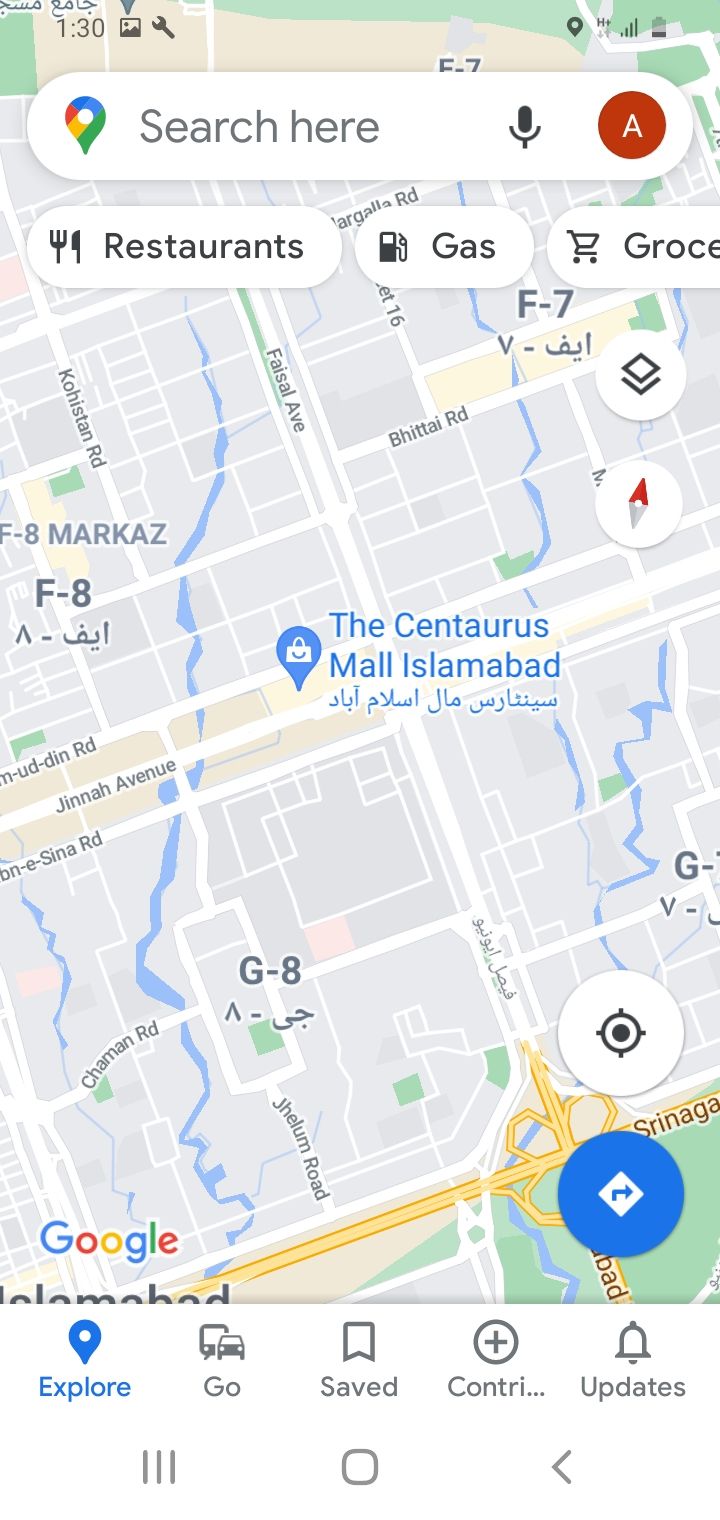This image shows a zoomed-in section of Google Maps displayed on a mobile device, focusing on a specific area around "Islamabad Mall." The map features a mixture of English and Arabic text, with an Arabic subheading adding an additional layer of information. "Islamabad Mall" is prominently pinned on the map, with some Arabic script appearing underneath this pin.

The layout highlights various city blocks spreading outward from the center focus on Islamabad Mall. Several streets are named, providing a detailed view of the surrounding area. 

At the top of the interface, the Google Maps search bar is visible, featuring a microphone icon that allows users to conduct voice searches. There are also quick-access buttons labeled "Restaurants," "Gas," and "Grocery" for convenient navigation to these essential services.

Towards the bottom of the screen, a menu provides options for "Explore," "Go," "Saved," "Contribute," and "Updates," giving users various functionalities to interact with the map and its data.